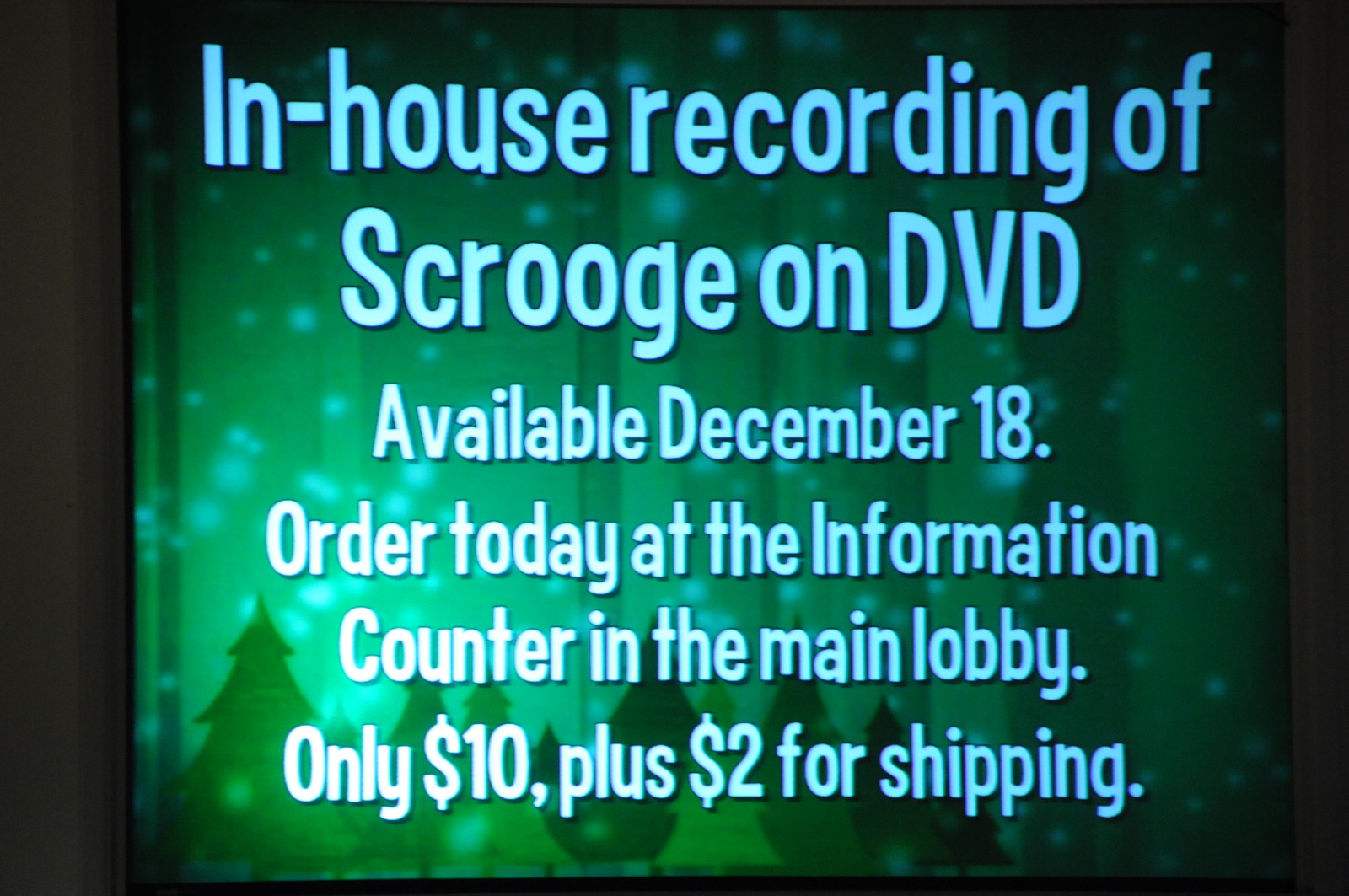This image is a wide rectangular digital poster featuring a festive advertisement for the in-house recording of "Scrooge" on DVD. The background is a gradient of green, brighter on the left side, accompanied by light blue text with dark borders. The text reads, "In-house recording of 'Scrooge' on DVD. Available December 18. Order today at the information counter in the main lobby. Only $10 plus $2 for shipping." The background theme includes a sky filled with snowflakes, depicted as pale green polka dots, falling against a serene, wintry scene of Christmas trees. The trees, drawn simply with triangular shapes, alternate in bright and dark green and gradually decrease in size from left to right. Black vertical lines frame the poster on both sides, adding to the detailed festive design.